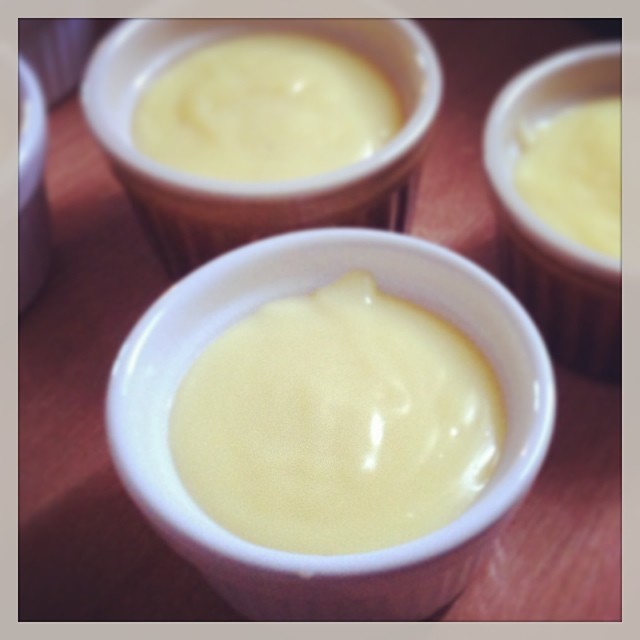The image displays a close-up of several white ramekins filled with a creamy yellow substance, likely vanilla pudding or a similar dish. The focus of the image is a prominently placed ramekin in the foreground, which takes up a significant portion of the frame. Above and to the left, another cup is visible with more yellow custard-like content. Additional ramekins are scattered towards the upper left and the upper right, with the ones at the top blending slightly into the background. The scene appears somewhat out of focus but clearly shows the items. A light source illuminates the cups, creating a shine on the custard and shadows around the dishes, all of which are set on a brown wooden table.